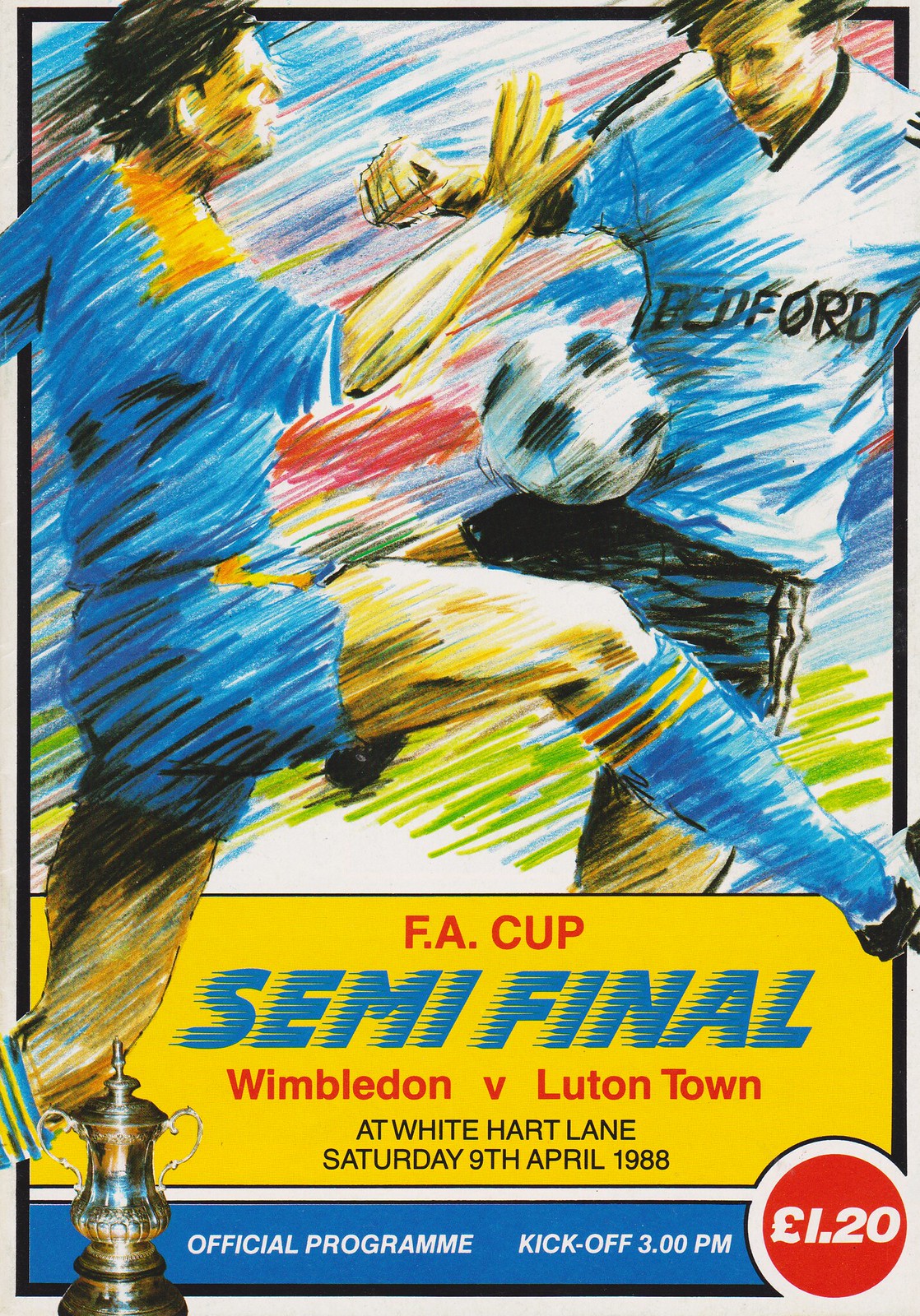This is a vividly illustrated program for the FA Cup semi-final match between Wimbledon and Luton Town, held at White Hart Lane on Saturday, 9th April 1988. The artwork prominently features two soccer players facing each other; one sports a blue jersey with blue shorts accented in yellow, while the other wears a blue jersey and dark shorts with black accents. A soccer ball is positioned between the players, and the entire illustration has a brushstroke or crayon-like effect, giving it a textured and dynamic appearance. 

Beneath this scene, a yellow banner with red and blue lettering announces the event specifics: "FA Cup" in red, "semi-final" in blue, and "Wimbledon versus Luton Town" in red. The details continue with "At White Hart Lane, Saturday 9th April 1988" in black font. In the lower left corner, there is a depiction of a trophy. A blue banner at the bottom of the program states, in white font, "official program, kickoff 3 p.m." Lastly, a red circle in the lower right corner indicates the cost of the program, "£1.20," in white and red.